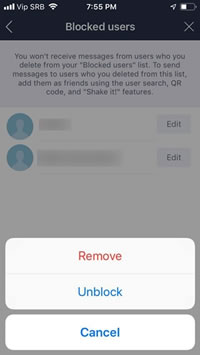The image is a smartphone screenshot displaying a blocked users management screen. At the top left, the screen indicates full network strength with four white bars and the time, 7:55 PM. Adjacent to this, it reads "VIP, SRB, full range for sound." The top right corner shows the battery indicator, which is slightly less than half full.

Below this status bar, the interface features a left arrow icon and the title "Blocked Users" in white text, all set against a black background. On the right side of this header, there's a white "X" icon, likely for closing the screen.

Beneath the header, a gray box contains important information in darker gray text: "You won't receive messages from users who you deleted from your blocked users list. To send messages to users who you deleted from this list, add them as friends using the user search, QR code, or shake it features."

Following this informational box, the screen displays two user entries. Each entry consists of a generic graphic of a profile portrait inside circular icons, accompanied by a gray bar to the right and an edit key icon on the far right.

At the bottom of the screen, three options are presented in distinct sections: 
1. A white box with "Remove" in red text.
2. A white box with "Unblock" in blue text.
3. A final white box separated by a gray line stating "Cancel" in blue text.

The overall design employs a darker gray background and white symbols, providing functionality to manage blocked users with options to remove, unblock, or cancel actions.